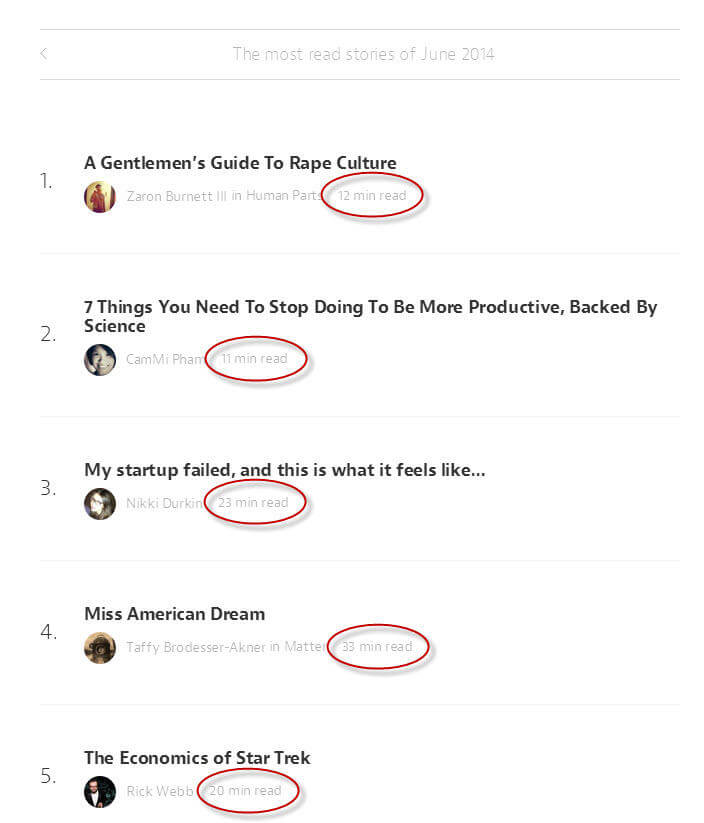Screenshot of a mobile website or app page displaying the "Most Read Stories of June 2014" category. A back arrow icon is present at the top left, allowing users to navigate to the previous category. 

Below the header, five stories are listed:
1. **"A Gentleman's Guide to Rape Culture"** by Zarin Burnett III in "Human Parts" – a 12-minute read. The read time is highlighted with a red oval.
2. **"7 Things You Need to Stop Doing to be More Productive (Backed by Science)"** read by Cammefam – an 11-minute read, also marked with a red oval.
3. **"My Startup Failed, and This is What It Feels Like"** by Nikki Durkin – a comprehensive 23-minute read, with the duration circled in red.
4. **"Miss American Dream"** by Taffy Brodesser-Akner in "Matter" – a lengthy 33-minute read, time circled in red.
5. **"The Economics of Star Trek"** by Rick Webb – a 20-minute read, with the read time circled in red.

The background of the page is entirely white, ensuring the text and red-circled read times stand out.